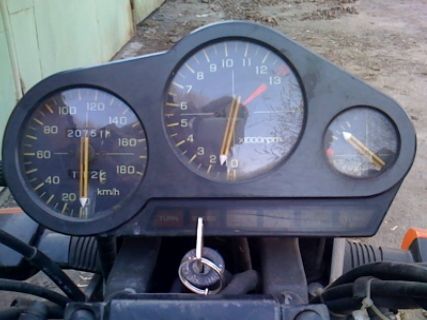This photograph captures the detailed view of a display panel on a machine or vehicle, likely an older model given the design. The panel itself is made of black metal or plastic and features three distinct dials. 

On the left, there is a circular speedometer with white numerals ranging from 20 to 180 kilometers per hour (KM/H). Each increment of speed is marked with lines for precise measurement. An odometer is positioned at the top of this dial, indicating the vehicle's total distance traveled.

The middle dial is another gauge of the same size, showcasing measurements from 0 to 13. The numerals are white but not entirely legible, and the gauge appears to have one or two hands, possibly used for measuring pressure or a similar parameter.

To the far right, a smaller, round gauge with a black face features a single hand and lacks numerical markings, which might indicate a simpler form of measurement, such as a temperature or pressure gauge.

Reflective surfaces on these dials reveal parts of a barren tree and the outline of a person's head, adding depth to the photograph. Below the dials, an ignition switch and a couple of black hoses are visible, providing further evidence that this display panel is part of a complex machine, likely a vehicle. The ground beneath the machine showcases a dirt surface, further situating this scene in an outdoor, perhaps rugged environment.